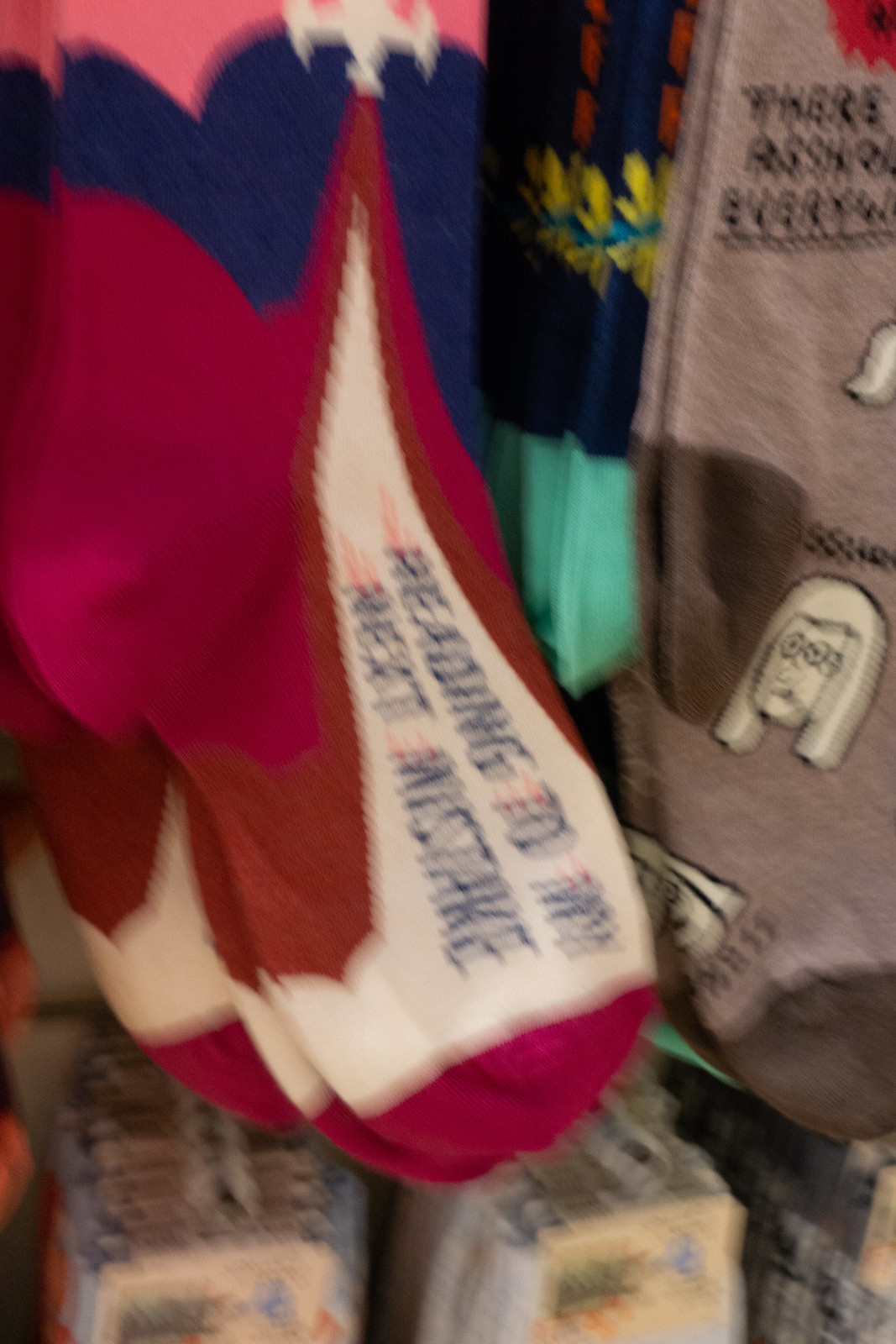In this very blurry photograph captured inside a store, an assortment of novelty socks hangs prominently from white hooks attached to display rods. The socks are neatly organized on shelves, with two particularly noticeable pairs at the top. One pair, which stands out the most, features a pink, blue, and red color scheme with a white stripe and a message in blue letters that reads, "Heading to my next mistake." This pair also displays what appears to be a ship motif between the pink and blue sections around the ankle. Adjacent to this is a gray pair adorned with an image of a woman's face. Despite the overall blurriness, the photograph depicts rows of vibrant, colorful socks with various designs and phrases, capturing the chaotic but charming essence of the store display.